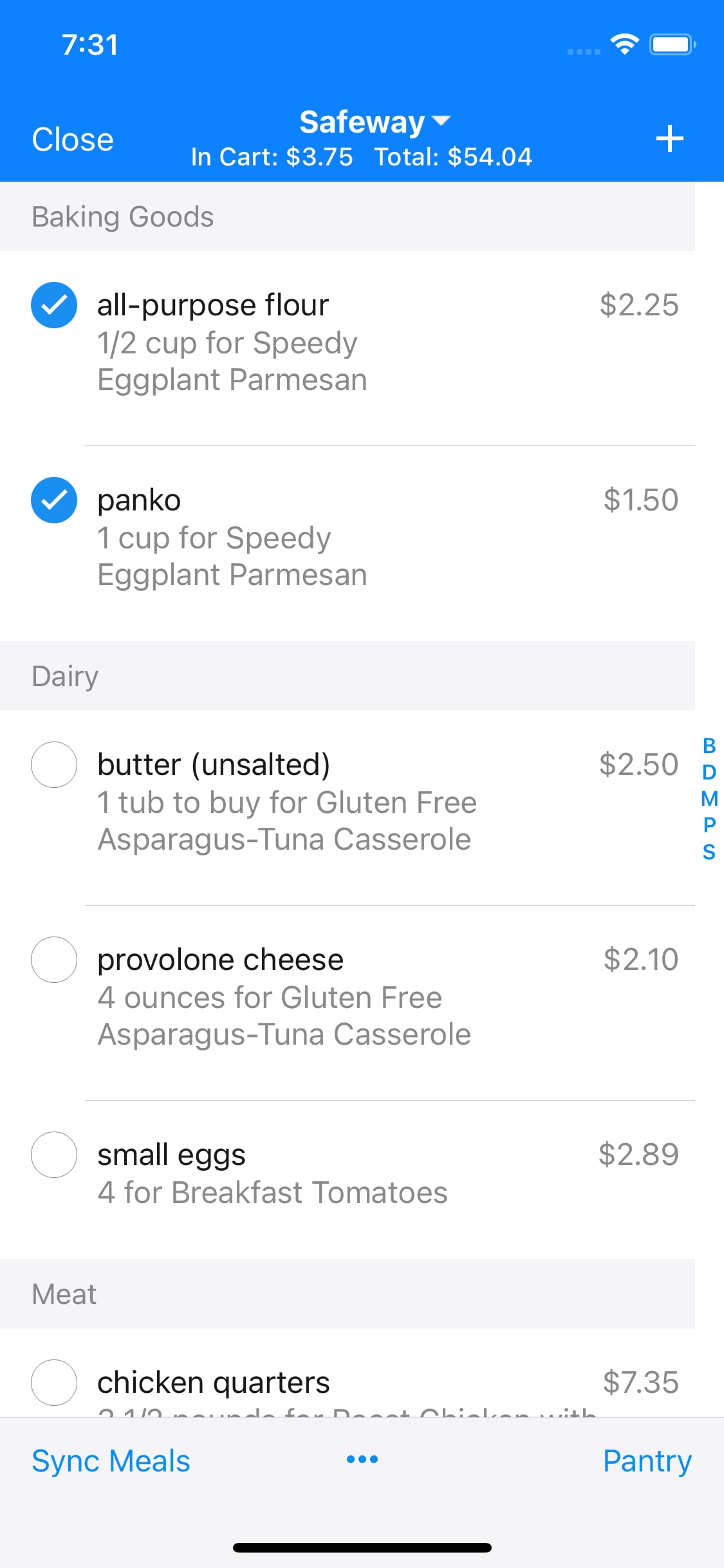This screenshot shows a smartphone interface, specifically a grocery shopping website for Safeway. The time in the top left corner indicates it's 7:31, and the battery icon shows it's nearly fully charged. The webpage prominently displays the Safeway logo at the top center.

In the visible contents, detailed listings under the Baking Goods category are shown. Items like all-purpose flour, priced at $2.25, and Panko, priced at $1.50, are marked with blue check marks indicating they have been selected. The item names are aligned on the left, while their prices are positioned on the far right.

Below, there are navigational tabs for different categories such as Dairy and Meat. Under the Dairy section, examples like Butter are listed, and the Meat section includes items like Chicken Quarters. The cart summary in the bottom right shows a total of $64.84 for 37 items. This detailed snapshot reflects a typical online grocery shopping experience through Safeway's mobile website.